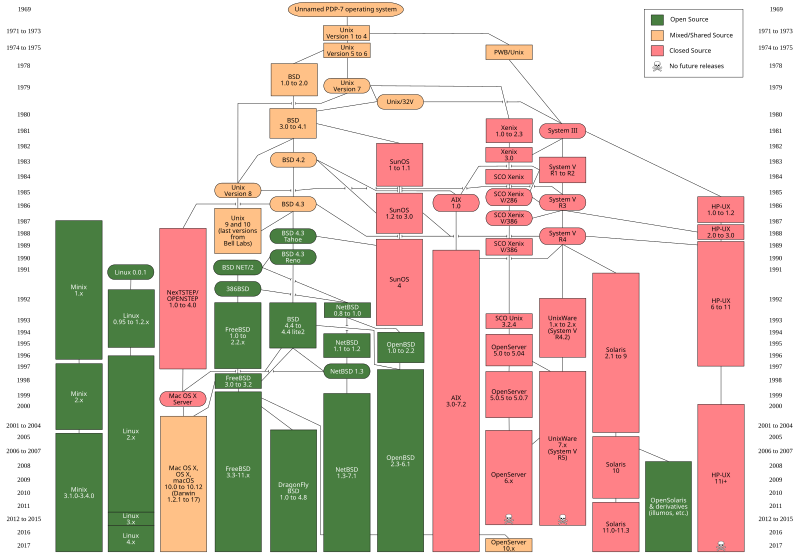This intricate diagram serves both as a timeline and a flow chart, illustrating the evolutionary path of various operating systems from 1969 to 2017. Years are marked on both the left and right sides of the chart, creating a mirrored timeline that tracks the progression year by year. At the top of the chart, we see the inception point labeled "unnamed POP7 operating system."

Below this, the chart documents the development of Unix, beginning with versions 3 to 4, then 5 to 6, and subsequently branching out in numerous directions. Overall, the chart features about 13 distinct columns and approximately 30 different squares and branches, each representing different operating systems or versions. These are color-coded to indicate their source type: green denotes open-source systems, peach represents mixed or shared source systems, and pink signifies closed-source systems. 

Additionally, several entries are marked with a skull icon, indicating that no future releases are expected for those particular versions. Notably, many of the pink (closed-source) entries include this skull symbol at the bottom. The detailed structure and color-coding provide a comprehensive overview of the complex development and diversification of operating systems over nearly five decades.